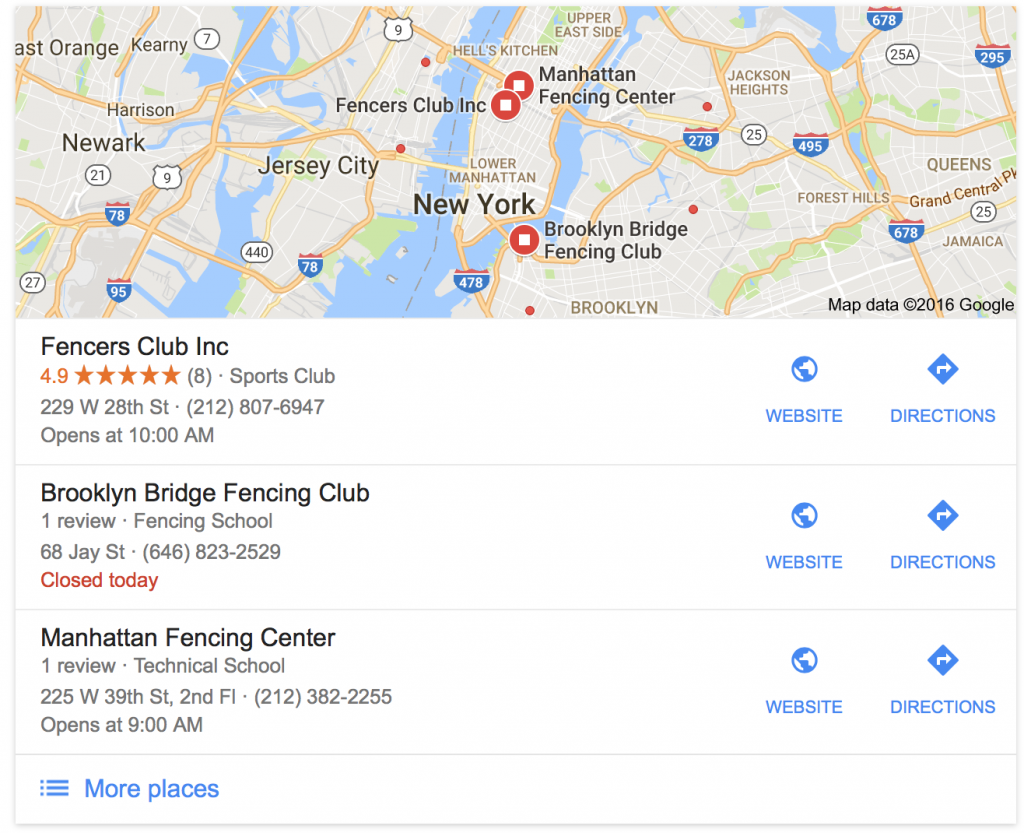This image is a detailed screenshot from Google Maps, prominently displaying the metropolitan area of New York City, including parts of Brooklyn and Manhattan. To the left, areas of New Jersey and Newark are also partially visible. The map is marked with several orange lines, possibly indicating major roads or transit routes, crossing through various parts of the city. 

In the central section of the map, three red circles with squares inside highlight specific locations, each labeled with black text to the right. At the top, the label reads "Manhattan," followed by "Fencing Center" beneath it, and finally "Brooklyn Bridge Fencing Club" at the bottom.

Below the map, three white rectangular boxes are arranged in separate rows, each containing information about fencing clubs. The first box on the left lists "Fencers Club, Inc." in black text, featuring five orange stars with a rating of 4.9 to the left and including the address and operational hours below. The second row highlights the "Brooklyn Bridge Fencing Club" with one review noted in light gray text, labeled as a "Fencing School," along with the address. The third row features the "Manhattan Fencing Center," also with a single review, described as a "Technical School" with its address provided.

At the bottom left of the image, light blue text indicates a link labeled "More Places." Adjacent to this link are three vertically stacked dots followed by three horizontal lines, likely representing menu options. Each row also contains buttons on the right side: the first being a "website" button and the second a blue "directions" button.